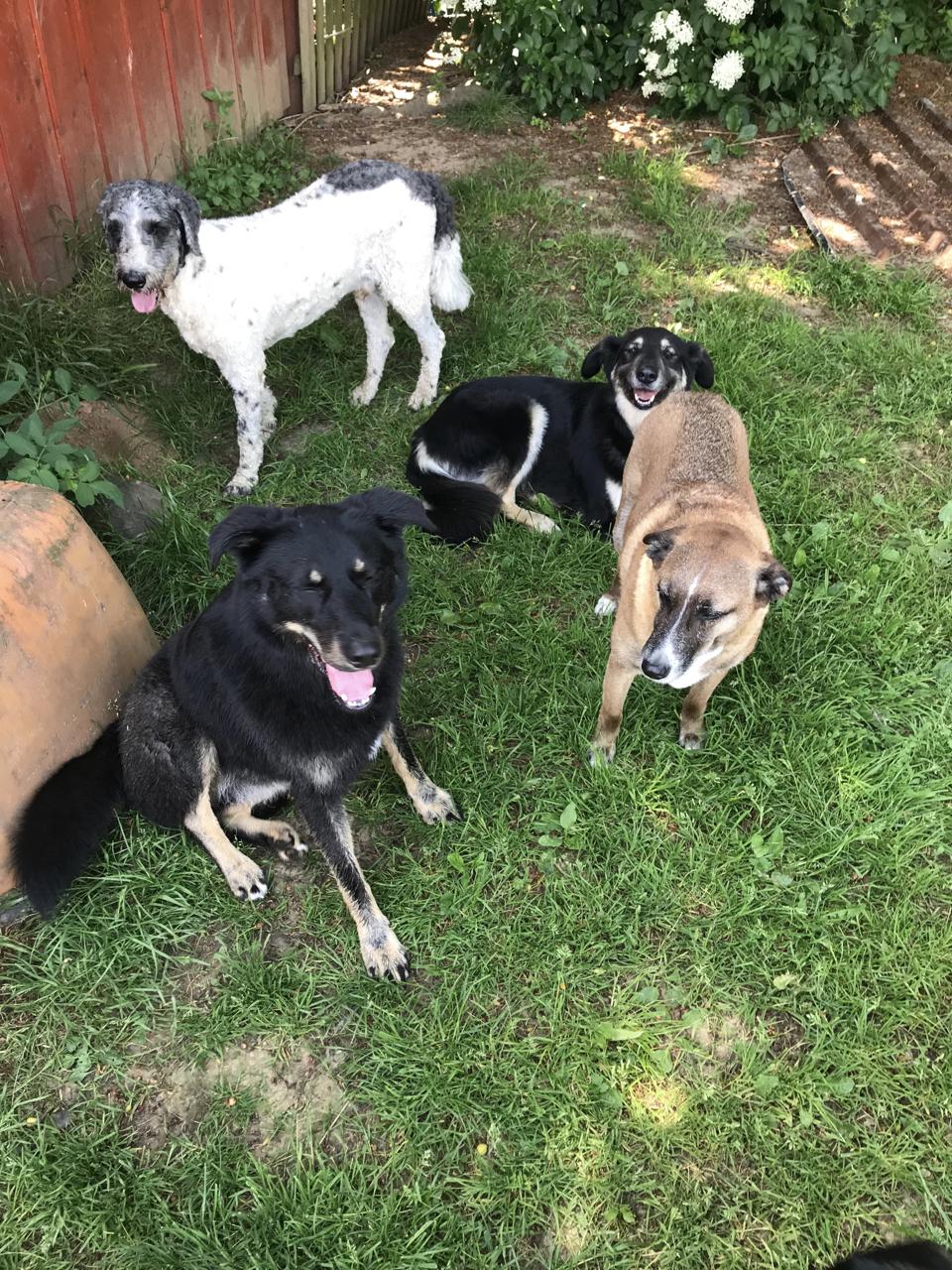A vibrant, color photograph captures a lively backyard scene featuring four joyful dogs on the lush grass. The perimeter is defined by an aged, red fence with patches of green mold, presenting a rustic charm. At the rear, shallow steps lead to a big, verdant bush adorned with beautiful white flowers.

To the top left, a predominantly white dog is easily noticeable due to its gray head and a distinctive black splodge on its back near the tail. This dog, like most, has its pink tongue lolling out happily. Directly counterclockwise from it, and sitting down, is a mostly black dog with sandy paws and a beige-brown underbelly. Its front legs and neckline bear similar beige hues, and it sits in a relaxed manner. 

Close to this dog, another sits with its hind legs down and front paws propped up, leaning casually against an orange object. This dog is also mostly black with two distinct brown spots above its eyes, and it shows off a happy expression with its mouth open and tongue out. Nearby, a fourth dog stands out with its sandy-colored body and black face, appearing energetic with short ears, displaying a playful stance.

The dogs, two lying down and two standing, exude a burst of energy and camaraderie, truly enjoying their time in the green haven.